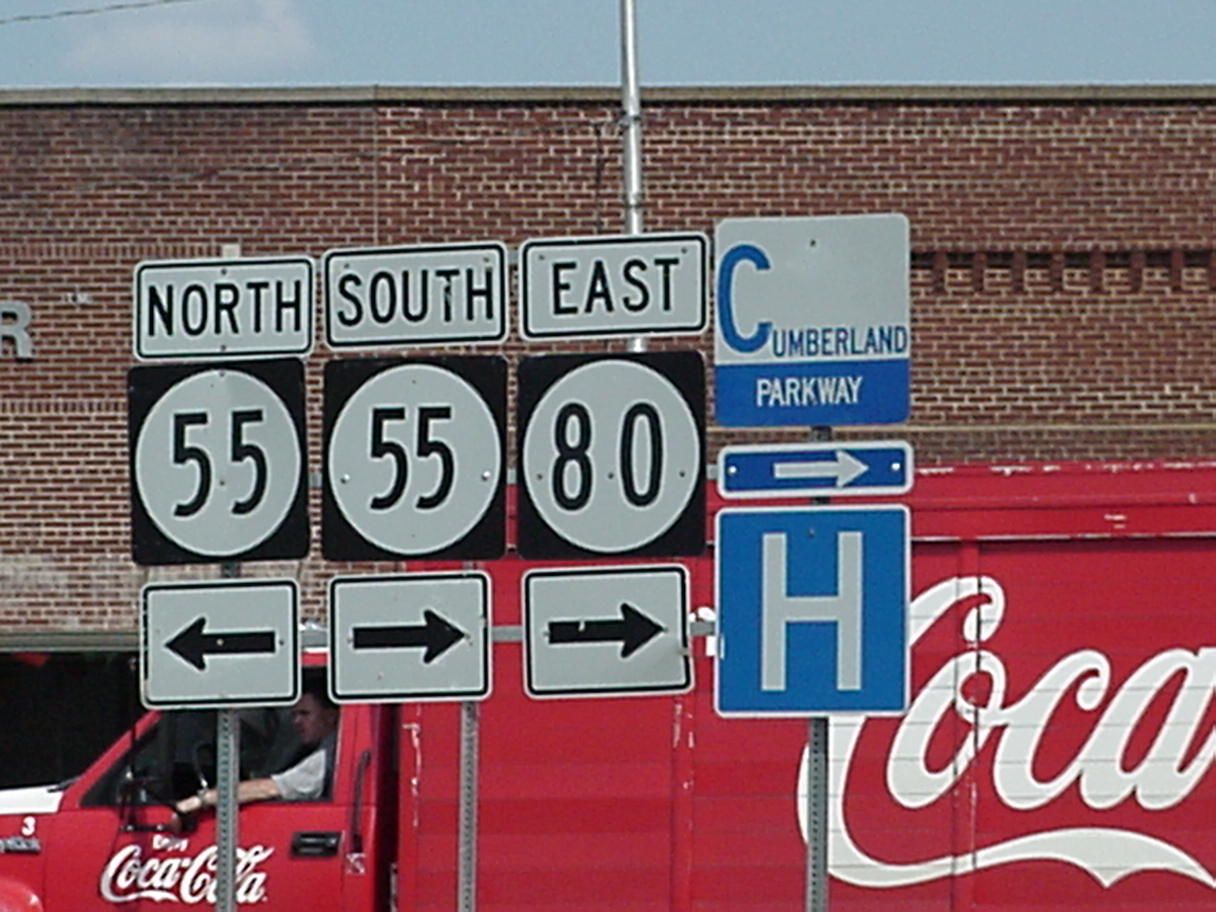This vibrant photograph captures a street scene featuring several directional signs and a prominent Coca-Cola delivery truck. In the foreground, there are three white and black highway signs in a horizontal line. The leftmost sign reads "55 North" and directs to the left, the middle sign reads "55 South" and directs to the right, and the rightmost sign reads "80 East" and directs to the right as well. Below the highway signs, there’s a blue and white sign indicating "Cumberland Parkway" with a right-pointing arrow, accompanied by a white "H" denoting a hospital to the right. In the background, a distinct red Coca-Cola truck is seen with a driver in a gray shirt visible through the cab window. The truck’s door is emblazoned with the white Coca-Cola logo. Behind the truck, a reddish-brown brick building adds an urban backdrop to the scene.